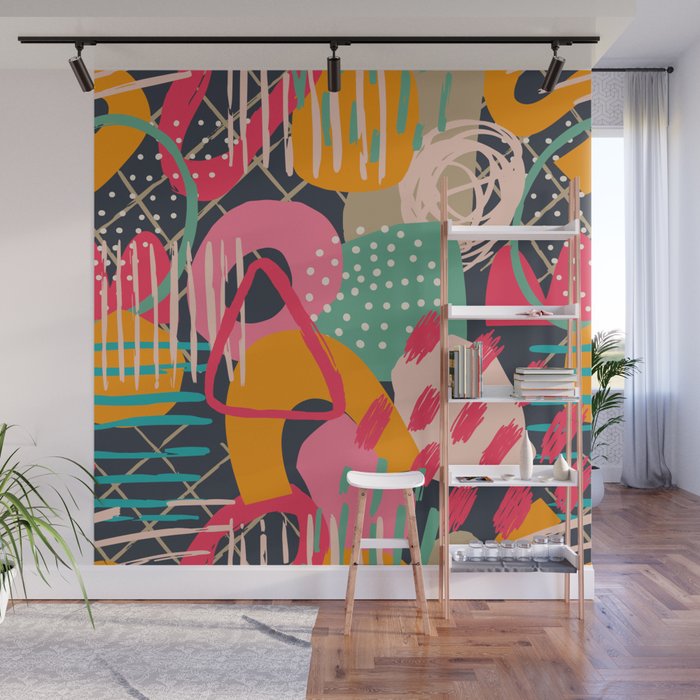This photograph showcases a well-decorated room that highlights an artistic mural painted onto a white wall. The mural boasts a vibrant, graffiti-style design with a plethora of colors including blues, yellows, pinks, greens, teal, and dark pink. The abstract painting spreads across most of the wall and features various shapes such as circles, triangles, U's, lines, dots, and dashes. 

The room itself has a distinctive wooden floor with a gray rug, adding a cozy touch. To the front left, a white pot houses a plant with long leaves, partially cropped out of the image. In front of the mural, there is a white stool with wooden legs and a five-tiered bookshelf with brown wooden legs and white shelves. This bookshelf holds cups, books, and assorted knickknacks, possibly suggesting an artistic workspace. 

The ceiling features a black metal bar equipped with three spotlights directed towards the mural, enhancing the visual impact of the artwork. The room also has white curtains and a partially open window on the right side, providing a subtle glimpse of the outdoors.